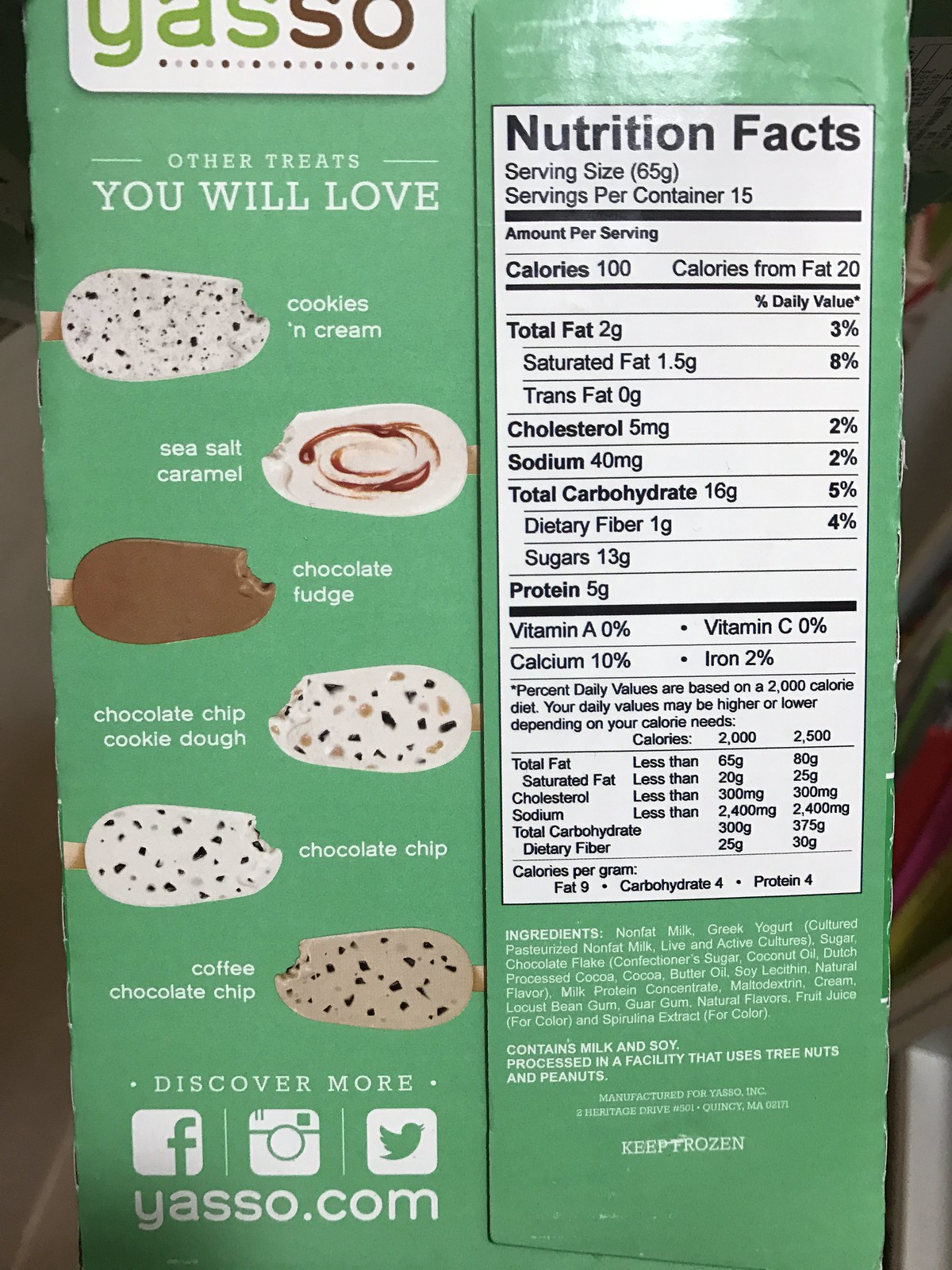The image features a detailed side view of a Yasso ice cream bar box, particularly focusing on its nutritional facts and variety options. The left section of the box prominently displays the Yasso logo at the top, followed by a list of other treats you might love: Cookies and Cream, Sea Salted Caramel, Chocolate Fudge, Chocolate Chip Cookie Dough, Chocolate Chip, and Coffee Chocolate Chip. Each flavor is accompanied by small pictures of the corresponding ice cream bars. The label also invites consumers to discover more, featuring icons for Facebook, Instagram, and Twitter, as well as the website yasso.com. The right side of the box, predominantly green, houses the nutrition facts in a white field with black text. The nutritional information provided includes serving size, calories, calories from fat, total fat, saturated fat, trans fat, cholesterol, sodium, total carbohydrate, dietary fiber, sugars, proteins, and various vitamins alongside their daily value percentages. At the bottom, it lists the ingredients and notes that the product contains milk and soy, and is processed in a facility that uses tree nuts and peanuts. The box is also marked with a "Keep Frozen" instruction and is manufactured for Yasso Inc., Eat Heritage Drive No. 501, Quincy, Massachusetts.